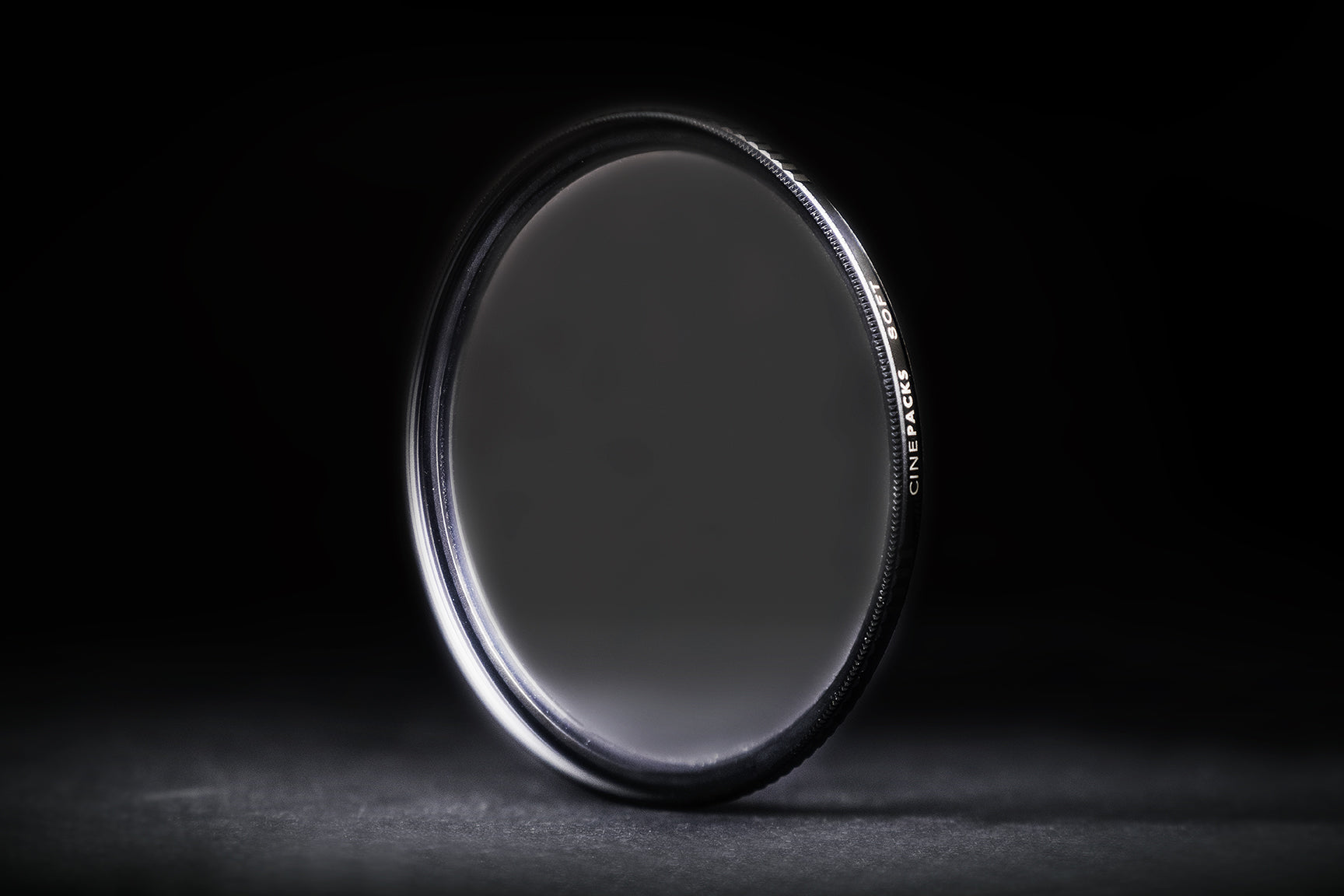This image depicts a close-up of a camera lens filter, standing upright on a dark grey surface. The background is completely black, providing a stark contrast. The filter features a frosty, mirror-like disc encased in a black metal ring. White text on the right side of the black ring reads "Cinepax Soft." The lens is slightly tilted, rotated about 40 degrees clockwise. The simplicity of the image highlights the lens filter as the central focus, with no additional elements or distractions present.